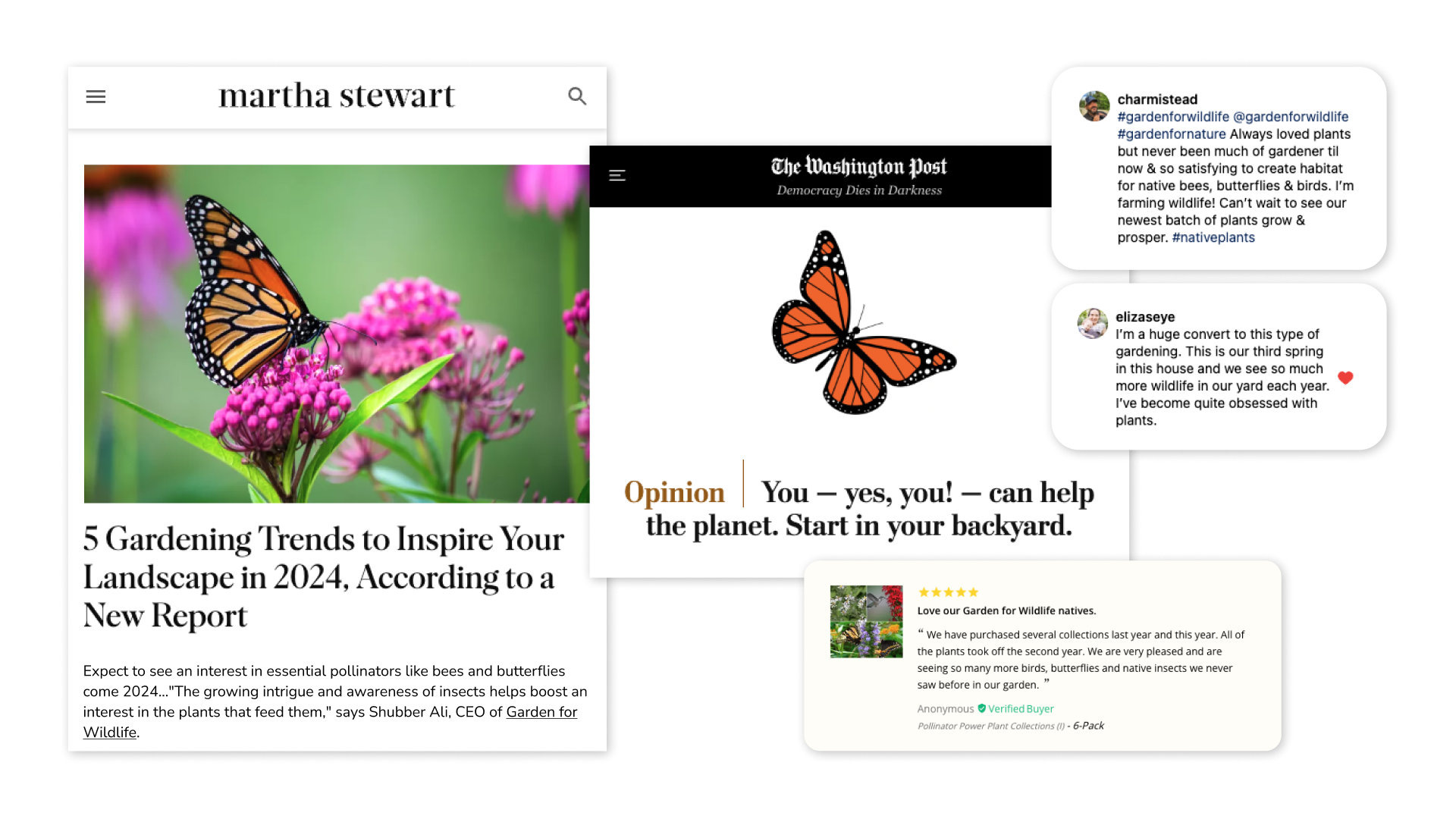The image is a detailed screenshot of a Martha Stewart website article titled "Five Gardening Trends to Inspire Your Landscape in 2024." Off to the left, there is a vibrant picture of a butterfly perched delicately on a purple flower. The article discusses emerging gardening trends and emphasizes the increasing appreciation for essential pollinators like bees and butterflies. According to Truby Alley, CEO of Garden for Wildlife, this growing fascination with insects highlights the importance of the plants that sustain them.

Next to this, there's another image featuring a screenshot of a Washington Post opinion piece titled "Yes, You Can Help the Planet, Start in Your Backyard." Below this, there's a five-star review, though the image and text are too small to discern clearly. Above the review, there are two social media comments. The first comment, from Facebook or Instagram, includes hashtags like #GardenForWildlife and #GardenForNature and reads:

"Always loved plants but never been much of a gardener till now and so satisfying to create a habitat for native bees, butterflies, and birds. I'm farming wildlife, can't wait to see our newest batch of plants grow and prosper. #NativePlants."

The second comment expresses a similar sentiment:

"I'm a huge convert to this type of gardening. This is our third spring in this house and we see so much more wildlife in our yard each year. I've become quite obsessed with plants. It's so satisfying to create a habitat for native plants."

This detailed screenshot captures the growing movement towards eco-friendly gardening practices and the collective enthusiasm for fostering habitats for essential pollinators.